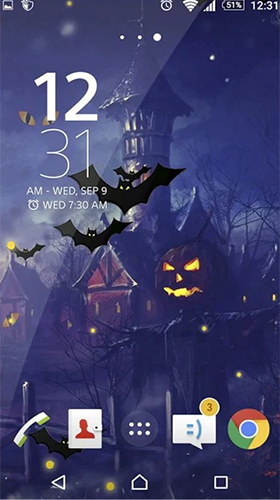This is a detailed screenshot taken in portrait mode, featuring a distinct Halloween-themed background that immediately sets a spooky tone. In the upper right-hand corner, the battery is at 51%, and the time reads 12:31 AM. Centrally, three navigation dots are present, with the third dot highlighted, indicating the current screen. To the left-center, the time is reiterated as 12:31 AM, with a date stamp of Wednesday, September 9th, and an alarm set for 3:00 AM the same day.

At the bottom of the image are the application icons: the Phone app, a likely Contacts app represented by a white icon, six dots symbolizing additional apps, an unknown app marked by an on-its-side emoji with three notifications, and the Google Chrome icon. 

Dominating the image is the Halloween-themed background, which features an ominous, haunted castle. The castle is dark and aged, with a hauntingly eerie roof. Central to the backdrop is a sinister jack-o'-lantern, with glaring eyes and a menacing mouth. Bats, depicted as black silhouettes with yellow eyes, ominously hover—particularly noticeable curving upward toward the top of the castle on the left side. Near the number 12 in the upper-left section of the screen are ghoulish yellow eyes with black pupils peering through the darkness, adding to the eerie atmosphere of the scene.